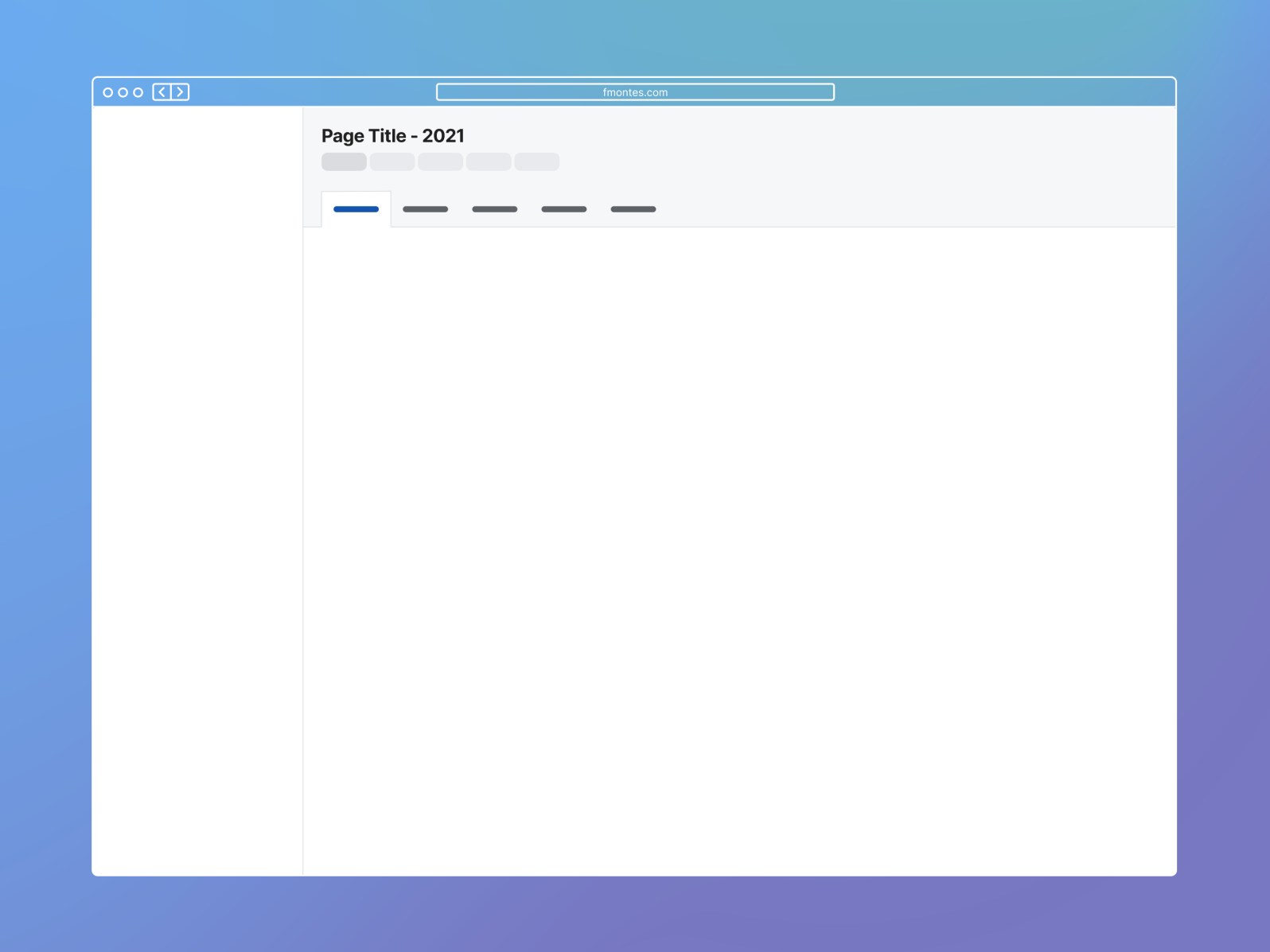The image features a rectangular layout with a light blue border enclosing a white page. In the upper left corner of this white page, there's a narrow blue border containing three circles and directional arrows pointing left and right. The top center of the white page displays the text "fmontes.com" in small white font on a blue banner. Below this banner, the main white page showcases black text that reads "Page Title 2021." Beneath this title are five light gray boxes, with the first box slightly darker than the others. Underneath the darker gray box, a blue line spans horizontally, revealing a tab that opens up another white page. To the right of this blue line, there are four horizontal dark gray lines.